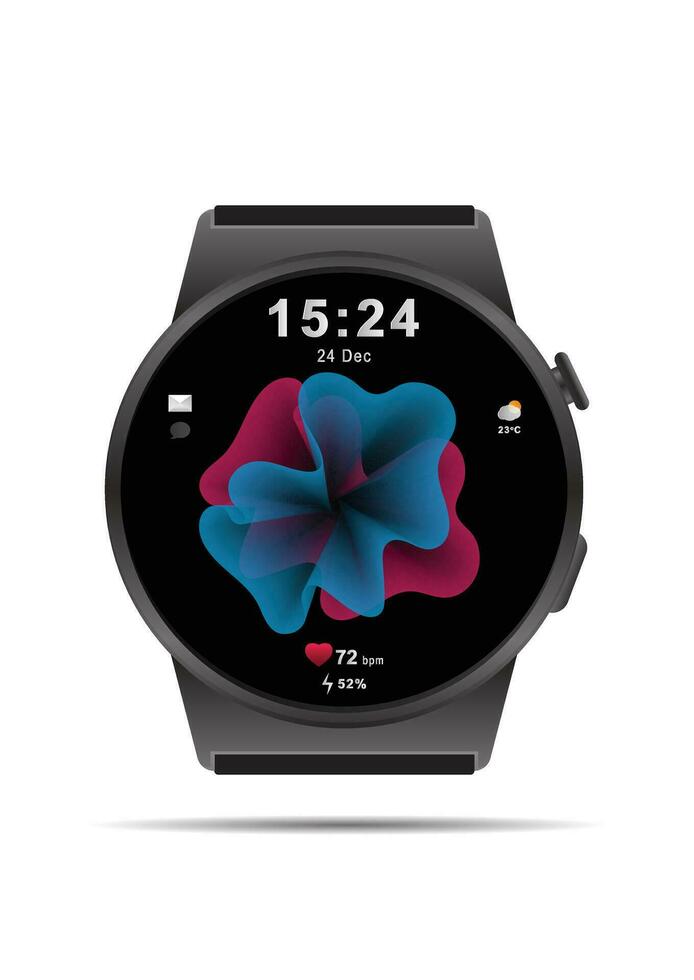This image features a detailed rendering of a dark gray smart watch, centered against a completely white background. The watch face is round with a black backdrop, bordered by a thin black trim and accented with silver edges. It features two buttons: a rounded one on the right side and a more rectangular one at the bottom right.

The LCD display prominently shows the time at 15:24 in white lettering at the top, followed by the date "24th of December." At the top left corner is a notification icon that appears to be for email, while the weather icon in the top right corner indicates partly sunny with a temperature of 23 degrees Celsius. The center of the display features a virtual flower-like design with blue and red coral-like patterns. Below this, a red heart icon displays "72 BPM," indicating the wearer’s heart rate, and a white lightning bolt icon indicates the battery life at 52%. The overall aesthetic gives the impression of a high-resolution graphic rather than a physical watch.